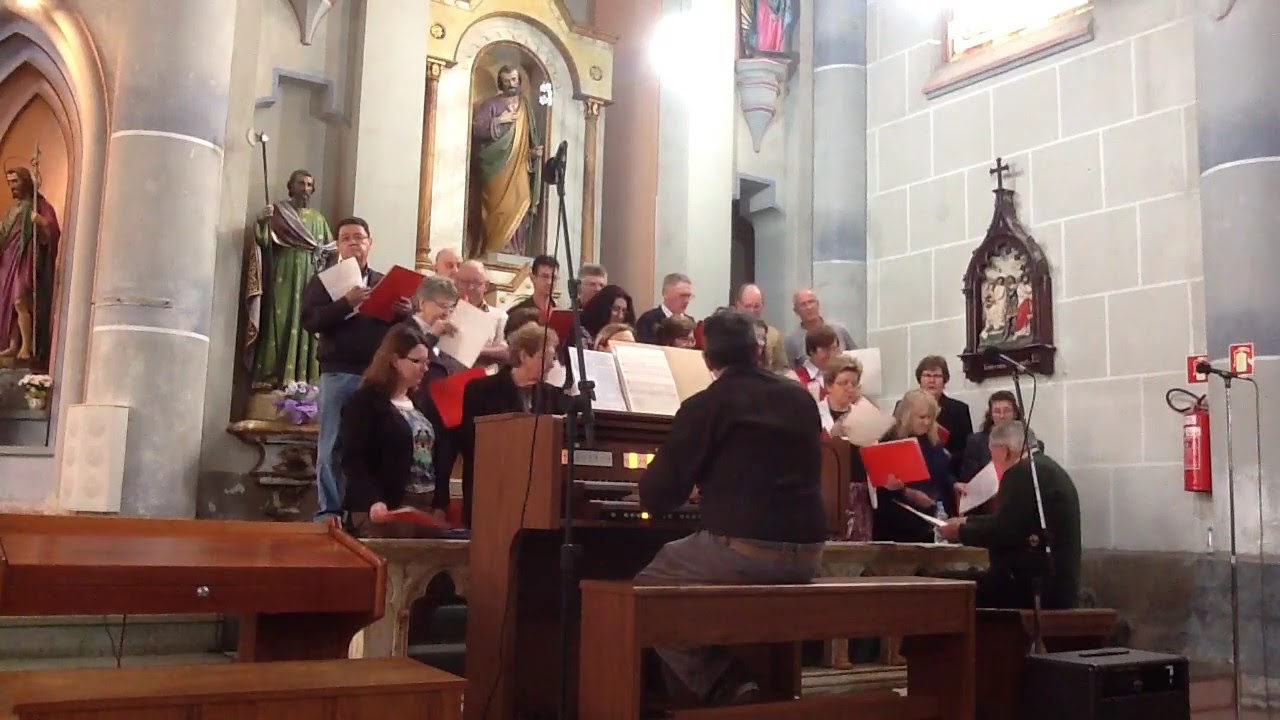This photograph captures a bright and ornate church interior, characterized by its gray stone walls and gold accents. The walls feature various colorful statues and altar pieces. In the foreground, a man dressed in a black long sleeve and gray pants is seated at a brown wood electronic organ, identifiable by its illuminated stops and yellowish tabs. The organ is flanked by several microphones and a red fire extinguisher is visible to the right.

Behind him, a choir of less than two dozen men and women stand on tiered platforms, each holding a red or orange folder. They appear to be practicing or rehearsing. The church is well-lit, enhancing the visual details of the architecture, including tiled columns and gold ornate arch inlets with statues. The setting conveys a reverent atmosphere filled with the anticipation of music.